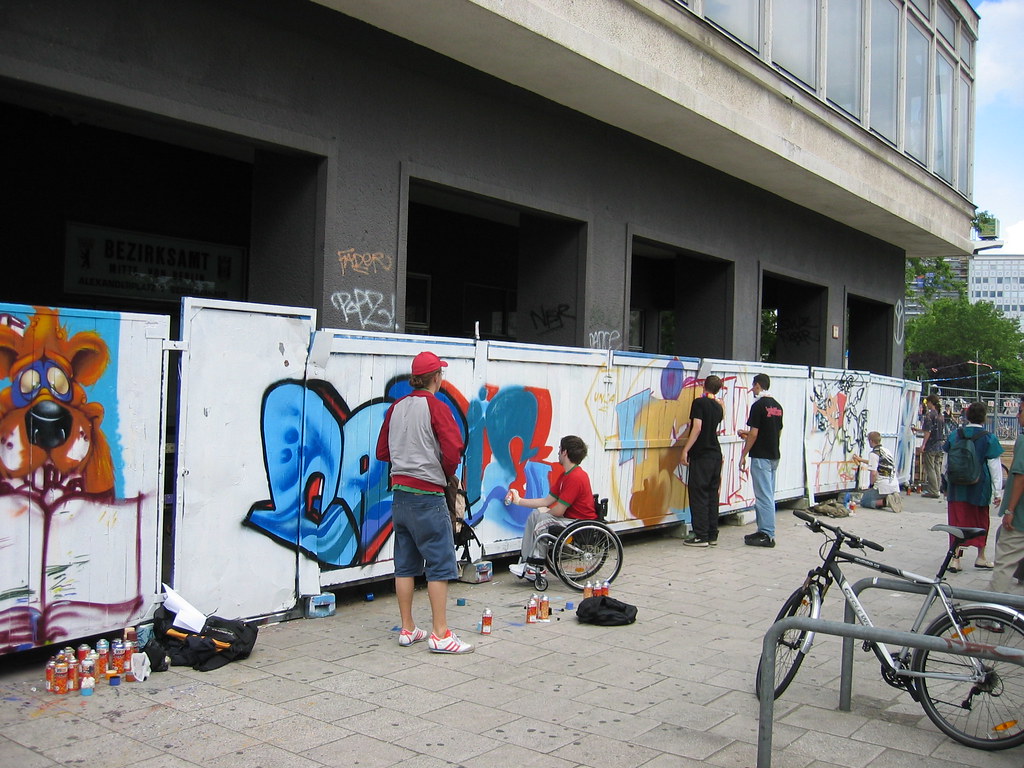This photograph captures a lively scene of several young artists engrossed in a graffiti art project on a large white wooden fence, possibly in a park or urban area. Central to the image, a man with a red baseball cap, a gray and red jacket, and short blue jean shorts stands near a man in a red shirt and gray pants who is in a wheelchair. This man in the wheelchair is actively involved in the project, applying red paint to the fence using a can of spray paint. Towards the left, two men wearing black t-shirts are absorbed in their work; the one on the left paired with black pants and the one on the right in light blue jeans, collaborating on a brown painting. In the background, a man in a white t-shirt is painting a section of the fence yellow, while another individual with long brown hair and a short blue t-shirt works with blue paint. The scene is bustling with artistic activity, including various cans of spray paint scattered around and even a bicycle situated in the bottom right corner. One panel of the graffiti notably features a cartoon dog, contributing to the diverse and colorful array of artwork covering the fence. People in the background watch with interest, adding to the vibrant community atmosphere of the scene.